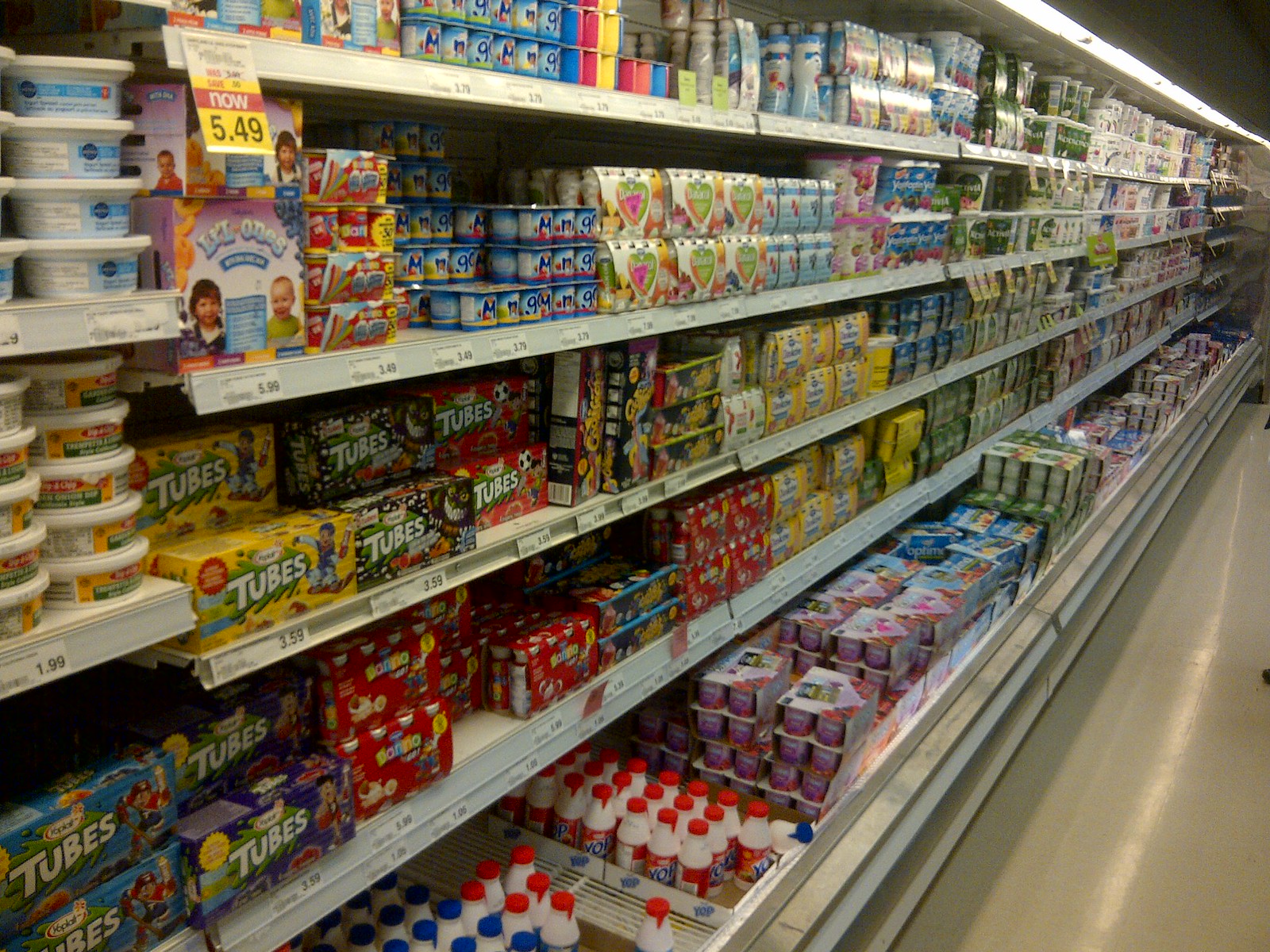This photograph captures a well-stocked aisle in a grocery store dedicated to yogurt, taken from an angle looking down the aisle. The shelving unit on the left side, stretching into the distance, is filled with a variety of yogurts displayed in a cooler-type shelving system. The metal shelves hold an assortment of yogurt products in various packaging, including large tubs, drinkable yogurts in bottles with blue and red caps, and boxes of tube yogurts in blue, purple, red, yellow, and green packaging. The bottom shelves prominently feature racks of drinkable yogurt bottles, some in six-packs and eight-packs encased in cardboard. The consistent fluorescent lighting from the ceiling illuminates the white tile floor that extends along the right-hand side. A clear path leads to the end of the aisle, with sales tags, including one notably advertising a "$5.49" price, affixed to some of the shelves. The upper right corner of the image shows a contrast of brightness from a beam of light and a small section of the black ceiling background, providing depth to the photograph.